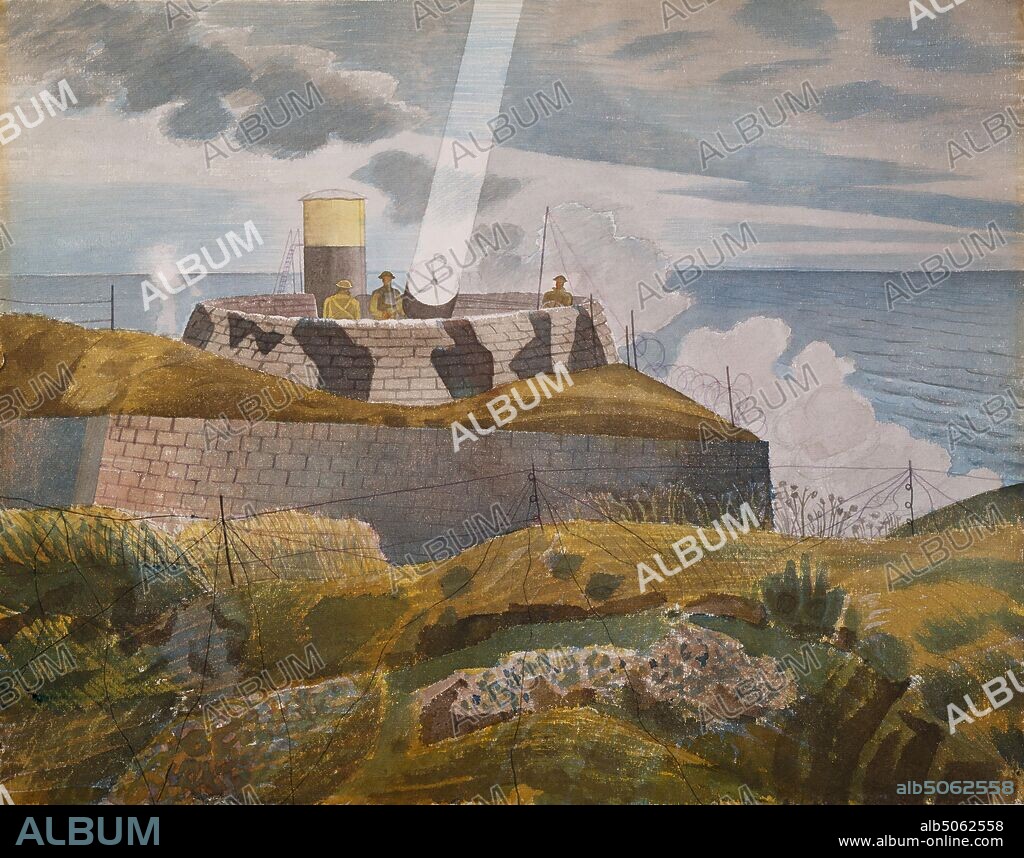This detailed painting depicts a sea fortress reminiscent of a World War II bunker, situated along a rugged shoreline with waves crashing against the shore and swirling foam. Dominating the scene is a yellow and black water tower or spotlight structure, equipped with a staircase or ladder. Three soldiers stand vigilantly, gazing out from a lookout point that resembles the top of a lighthouse. Surrounding them are white brick walls, barbed wire fences, and scattered military items. The landscape features rolling brown hills in the foreground, giving way to a vast, cloud-filled sky with a blue horizon and the ocean beyond. The image is marked repeatedly with a watermark that says "album," and in the bottom left corner on a black background, it reads "album." In the bottom right, the code "ALB 5062558 www.album.online.com" appears.